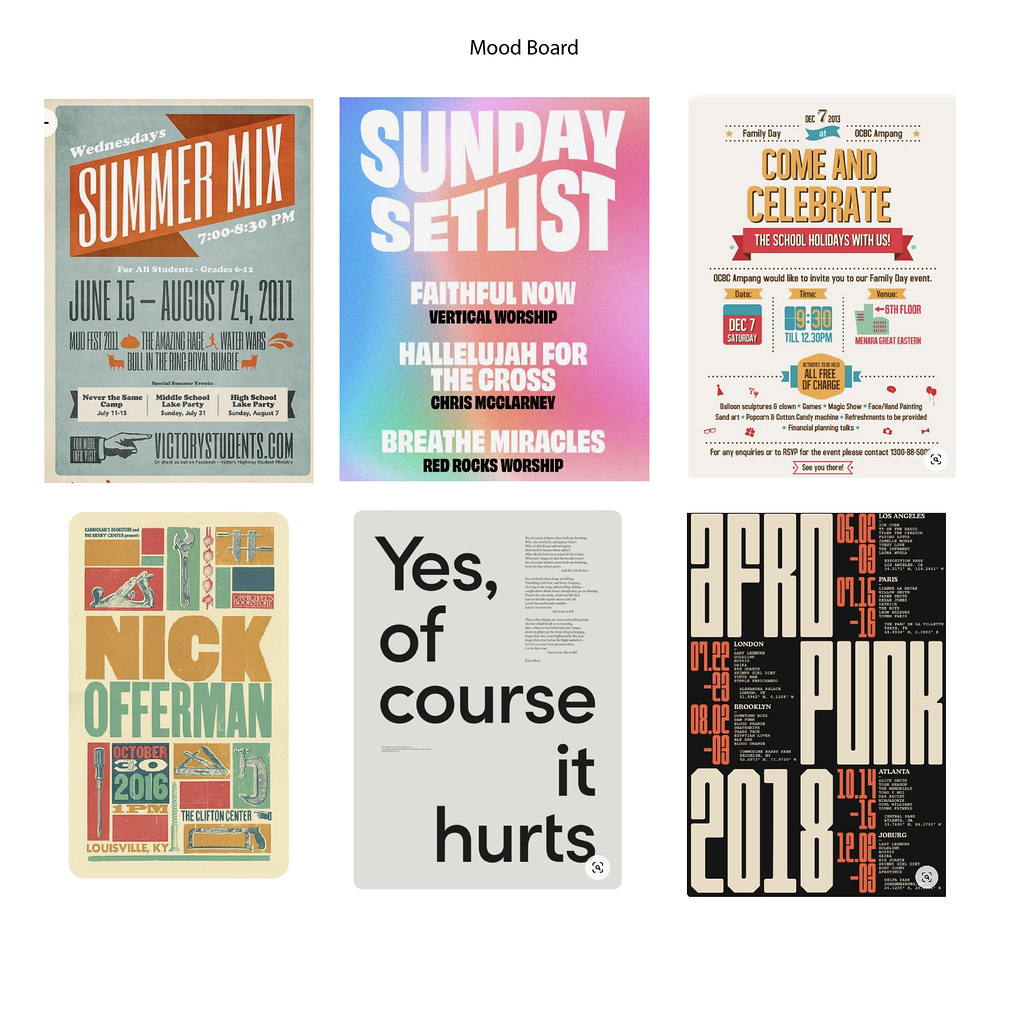The image displays a compilation of six vertical rectangular advertisements, each richly colored and distinct, likely related to musical events or celebrations. 

- **Top Left**: An ad with a gray background prominently featuring "Wednesdays" in white, followed by "summer mix" in bold white letters against an orange backdrop. The dates "June 15th-August 24th, 2011" are specified in large black text.
- **Top Center**: This colorful ad with a blue, green, coral, and dark pink gradient background announces "Sunday setlist" in curved, bold white letters. Additional text includes names and phrases like "Faithful now," "Vertical worship," "Hallelujah for the cross," "Chris McLarent," "Learn it," "Breathe miracles," and "Red Rocks worship."
- **Top Right**: Against a white background, it invites people to "come and celebrate" in orange letters. Further details, including dates, are present but too small to decipher.
- **Bottom Left**: Features "Nick Offerman" centrally, with "Nick" in brown block all-caps and "Offerman" in green all-caps. Surrounding the name are various colorful images.
- **Bottom Center**: A minimalist design on a white background with the phrase "yes, of course, it hurts" in black text; the first part is left-aligned while the word "hurts" is right-aligned.
- **Bottom Right**: This ad is marked by contrasting black sections and large white text. The layout reads "Afro" on the left, "Punk" centered to the right, and "2018" at the bottom left.

Overall, these advertisements, filled with vibrant color contrasts and bold texts, create an eclectic and visually stimulating mood board, seemingly focused on musical events and celebrations.